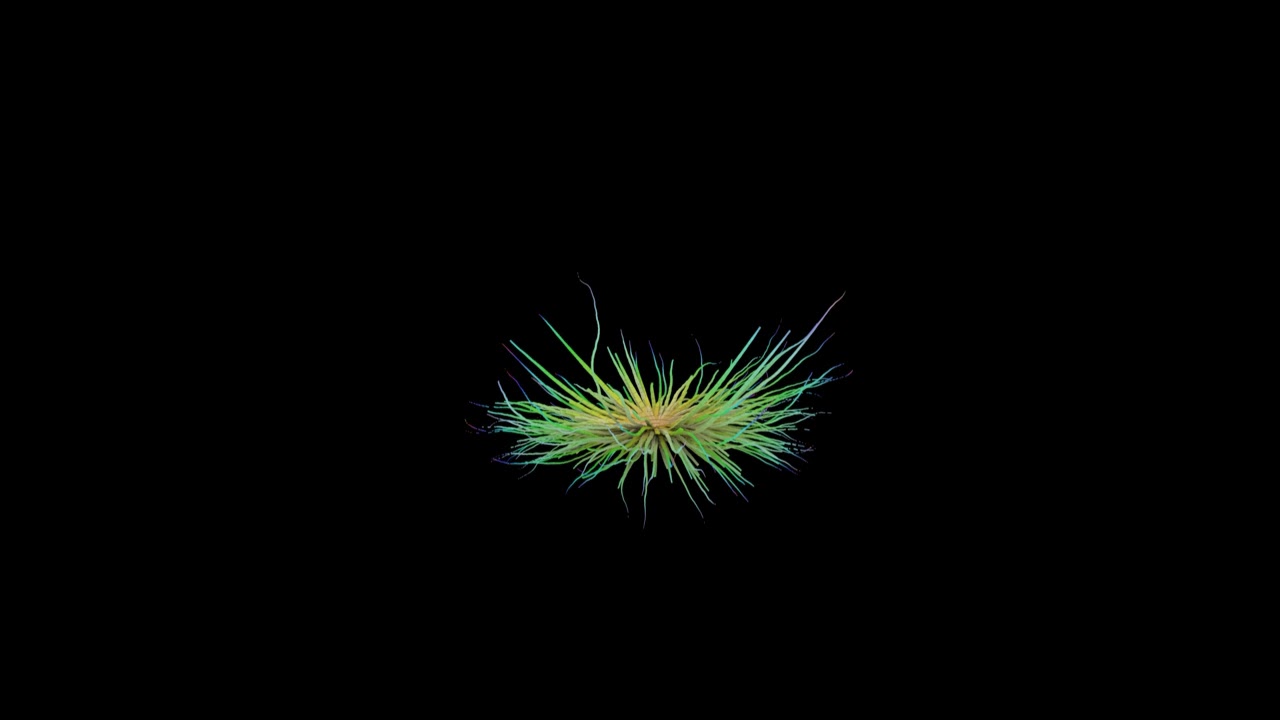The image features a digitally created, sea creature-like object centrally positioned against a flat, black background that covers 90% of the image. This mysterious object is small, potentially representing either a sea cucumber or a plant, with numerous thin, stringy tentacles extending in various directions—some long, some short, and of varying thickness. The object showcases a gradient of colors, predominantly white and yellow at its core, transitioning to hues of blue, green, and hints of red and tan towards its extremities. The intriguing, tentacle-like appendages give the impression of movement, although they remain stationary. The overall design makes the object appear to be floating in the darkness, with no other elements or text present in the frame.